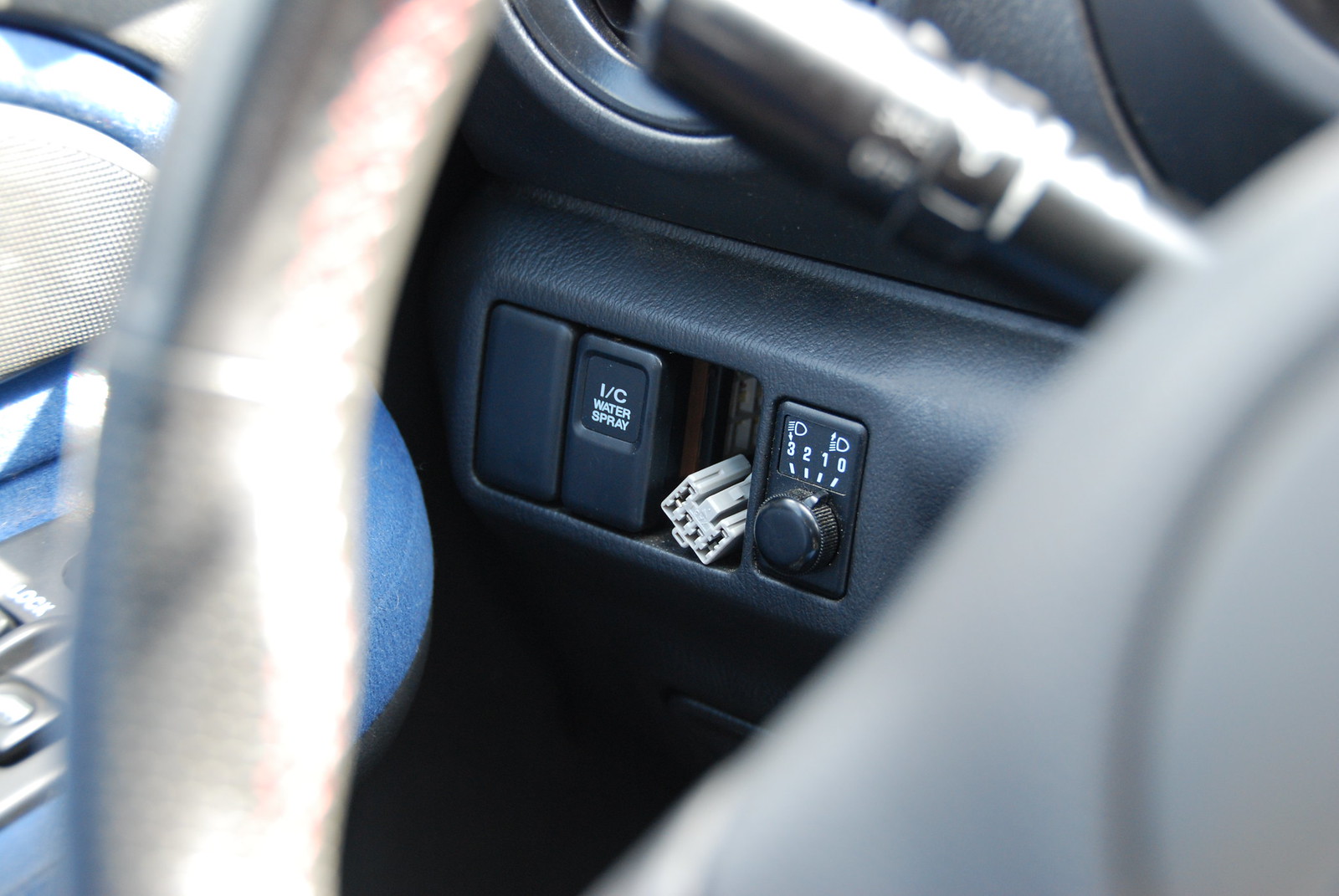Inside the car, the picture prominently features the left-hand side door panel and part of the dashboard console. On the door, the upper left corner houses a speaker, while the lower section is covered with a blue material. The door also has a panel equipped with controls for locking, window operation, and other functions. 

In the middle of the image, highlighting the dashboard console, there are several buttons. Notably, there is a plain button, a button labeled "I-C water spray," and a spot where a button is missing, revealing a white connector inside. Alongside these, there is a dial with settings numbered 0, 1, 2, and 3, likely connected to headlight operation, as indicated by the icons depicting headlights. The rest of the visible components, including the edge of the steering wheel on the right, are primarily composed of black plastic materials.